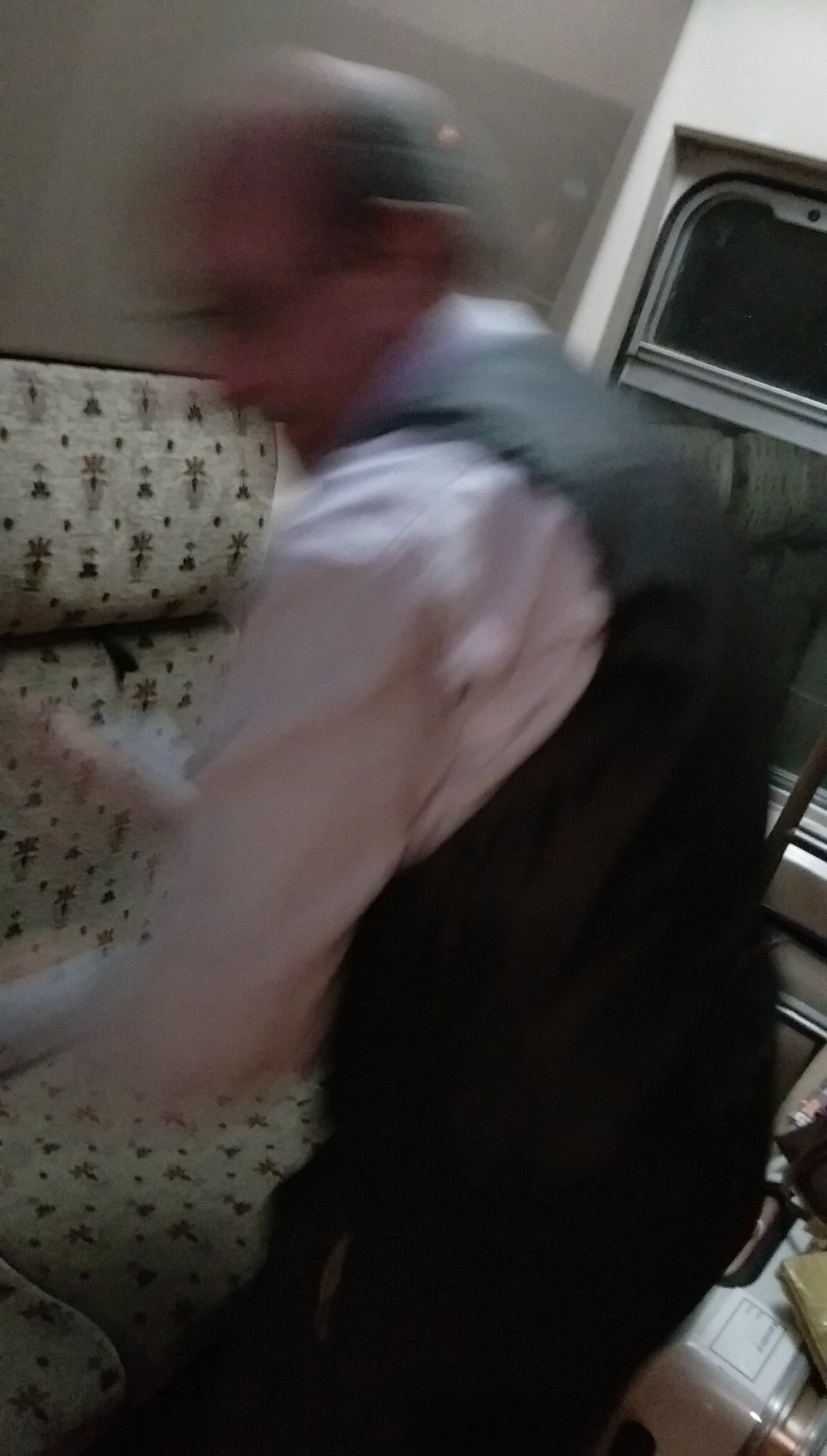A man, likely the bus driver, is seated on a bus, dressed formally in a white button-up shirt, black vest, and black pants. He wears glasses and exhibits a pattern of thinning hair with a mix of salt and pepper hues. The image is slightly blurry due to the man’s motion. He is captured leaning against a bus seat, which features a distinctive pattern resembling Chinese writing interspersed with dots. The fabric design includes alternating rows of complex characters and geometric shapes with dotted accents. Beyond the man, the upper part of a window is visible, showing the section where the window can be slid open. Part of the plastic armrest of the seat in front of him can also be seen.